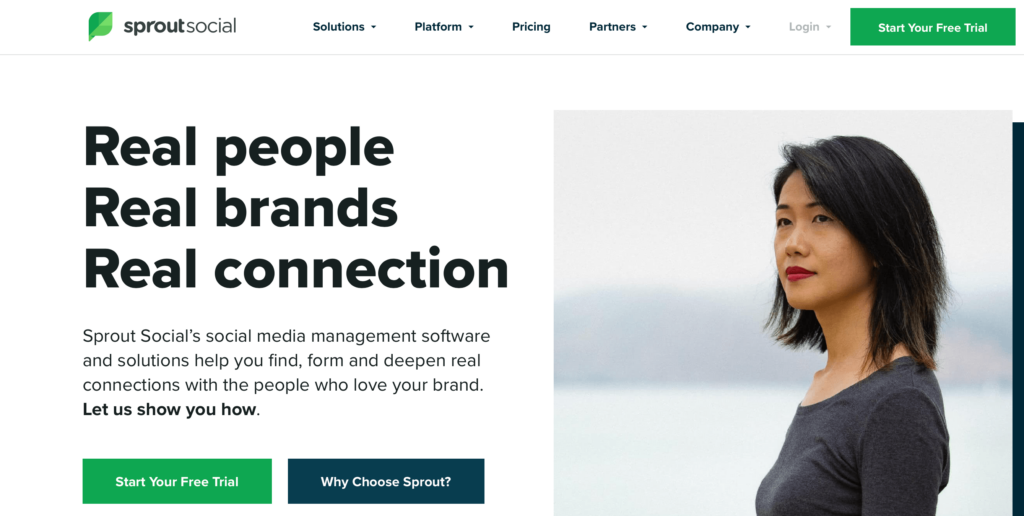The image depicts the homepage of Sprout Social's website, which prominently features its branding in the upper left-hand corner, including a green leaf icon. The navigation bar at the top offers links titled "Solutions," "Platform," "Pricing," "Partners," and "Company." To the far right of the navigation bar, there are options to log in or start a free trial, the latter clearly highlighted in a vibrant green button.

Centered on the webpage is the slogan "Real People, Real Brands, Real Connection," emphasizing the essence of Sprout Social's services. Below this motto, it elaborates that Sprout Social's social media management software and solutions aim to help users forge and deepen genuine connections with their audience. Below this text is another green button inviting visitors to "Start Your Free Trial," and a contrasting black button that says "Why Choose Sprout."

Dominating the right side of the main content area is an image of an Asian girl. She is dressed in a long-sleeve gray shirt and has neatly styled, shoulder-length black hair. Her face is serious, framed with red lipstick. She gazes off into the distance, seemingly lost in thought. The background behind her is blurred, displaying a natural landscape with a body of water—likely a lake—and distant mountains, further suggesting she is outdoors. The combination of the serious expression and the serene backdrop adds a contemplative mood to the image.